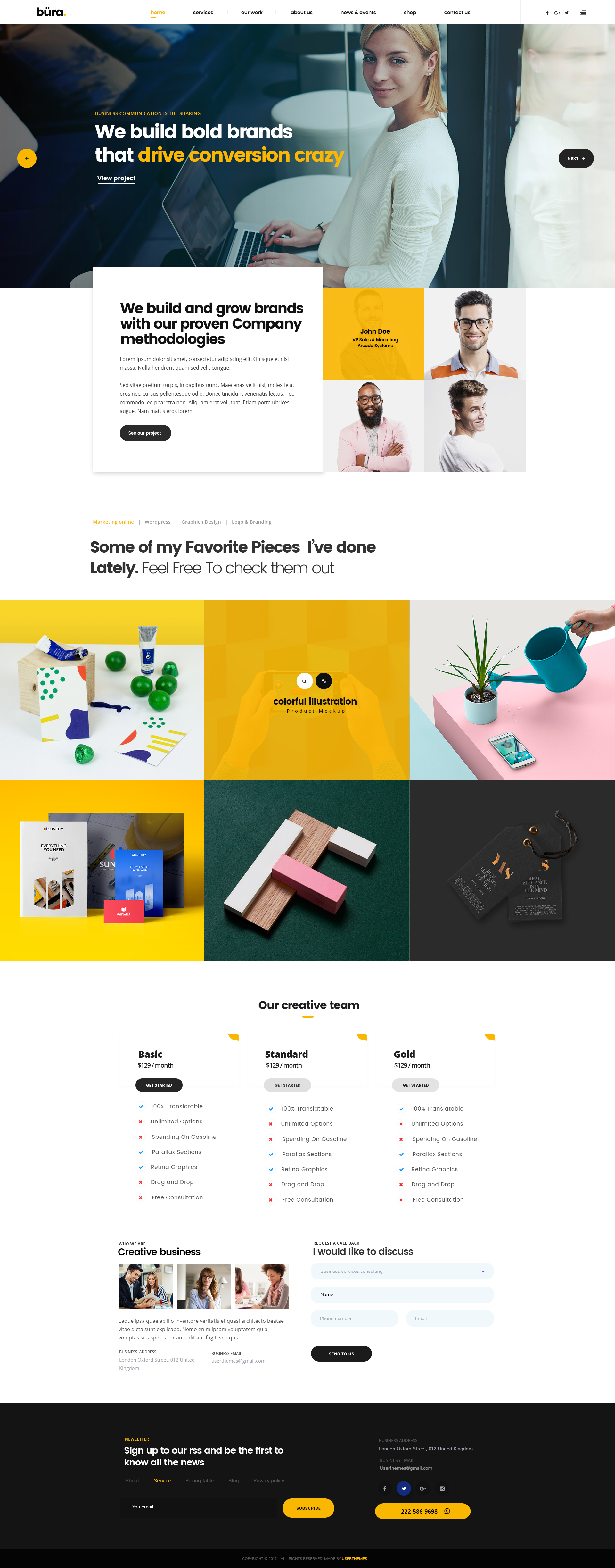The image appears to be a screenshot from an application called Bura, distinguished by the "ü" with umlauts. The app's name is displayed in the upper left-hand corner. The navigation bar across the top features options: Home (highlighted in yellow), Services, Our Work, About Us, News and Events, Shop, and Contact Us. On the right side of the bar, there are icons for Facebook, Google+, Twitter, and a menu icon.

In the main content area, there's a prominent image of a blonde woman wearing a white shirt, leaning against a pole or window, with a laptop on her lap. Overlaid on this image is the bold text, "We Build Bold Brands That Drive Conversion Crazy." Below this, another box contains the message, "We Build and Grow Brands With Our Proven Company Methodologies."

To the right of this message are four blocks. The first block has a blurred face with the text "John Doe, BP Sales and Marketing, Arcade Systems." Next to it, there's a picture of a man wearing glasses. Below these are two more images: on the left, a man with glasses, a beard, and a pink jacket; on the right, a clean-shaven man with short hair wearing a white T-shirt.

Further down is a section showcasing favorite projects, titled "Some of My Favorite Pieces I've Done Lately. Feel Free to Check Them Out." It includes five images: 
1. Little paintings displayed with green fruits resembling tiny peppers.
2. A colorful illustration in the middle.
3. On the right, a person watering a small dracaena plant.

Below these, there's a book-themed image titled "Everything You Need," showing four books, one of which is "Sun City: Everything You Need." 

Continuing down, there's an "Our Creative Team" section and subscription options: Basic, Standard, and Gold, all priced at $129 a month. Each option features a "Get Started" button, with the Basic option highlighted in black.

At the bottom, a sign-up prompt reads, "Sign up to our RSS and be the first to know all the news."